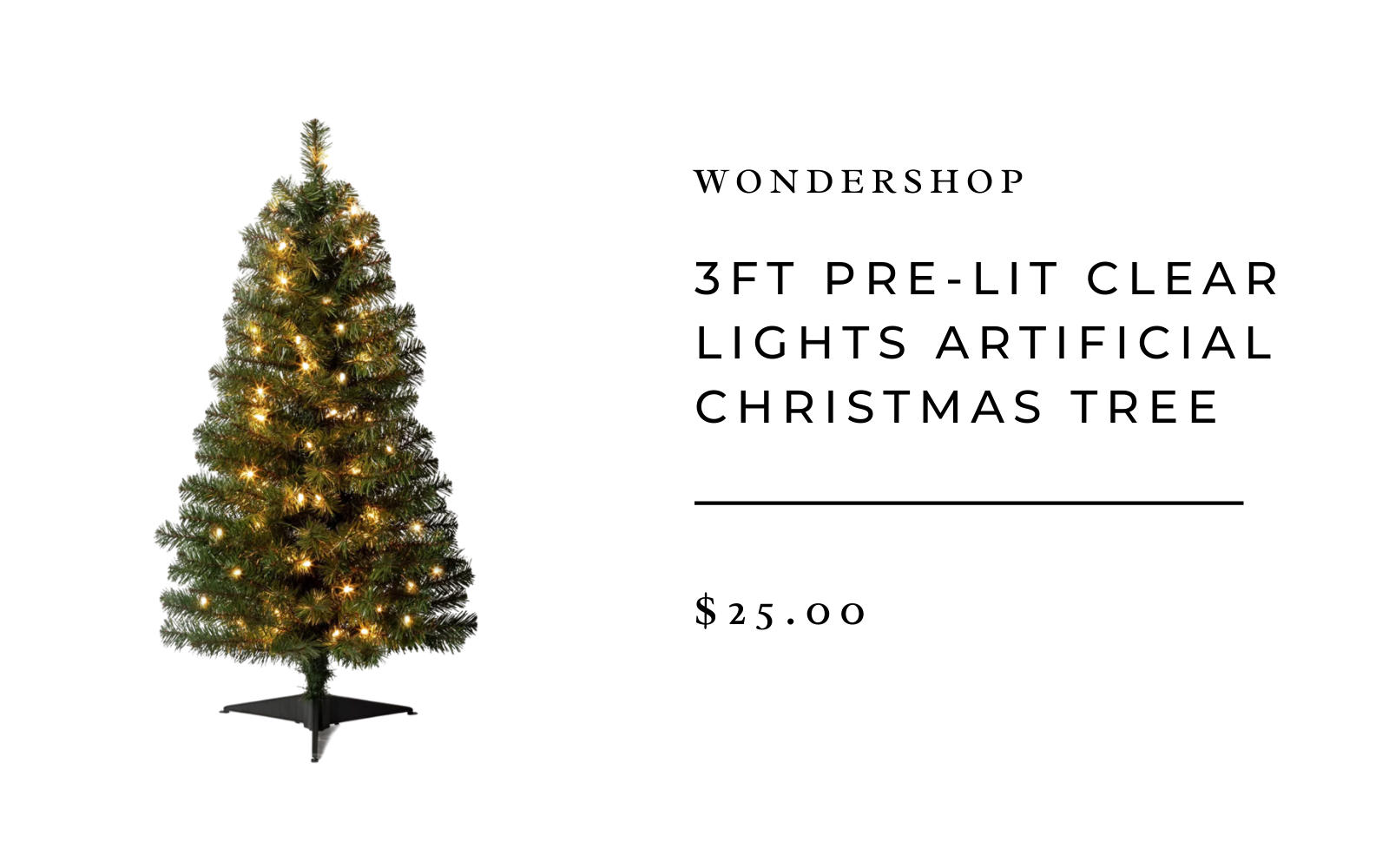**Wondershop 3-Foot Pre-Lit Clear Lights Artificial Christmas Tree - $25**

This detailed web page from Wondershop prominently features the product name in bold, all-capital letters at the center of the page. The product is a "3-Foot Pre-Lit Clear Lights Artificial Christmas Tree." Below the product name, a clear line separates the title section from the detailed product information. Listed at $25, the concise price is displayed in black text. 

The central visual attraction of the page is a stunning photograph of the tree, showcasing it in all its illuminated glory. The image captures a front-facing view of the tree adorned with clear lights, allowing potential buyers a clear perspective on its appearance. The tree stands on a sturdy base, with solid prongs extending out to support it. No ornaments are present, putting full emphasis on the elegant simplicity of the lights and the tree's natural design.

A noteworthy detail is a single branch at the top center of the tree, highlighted by an illuminating light. It seems the page is purely informational with no direct contact information or ordering options provided. Potential buyers are advised that the tree is available from Wondershop, even though further instructions on how to proceed with the purchase are not included within this web page.